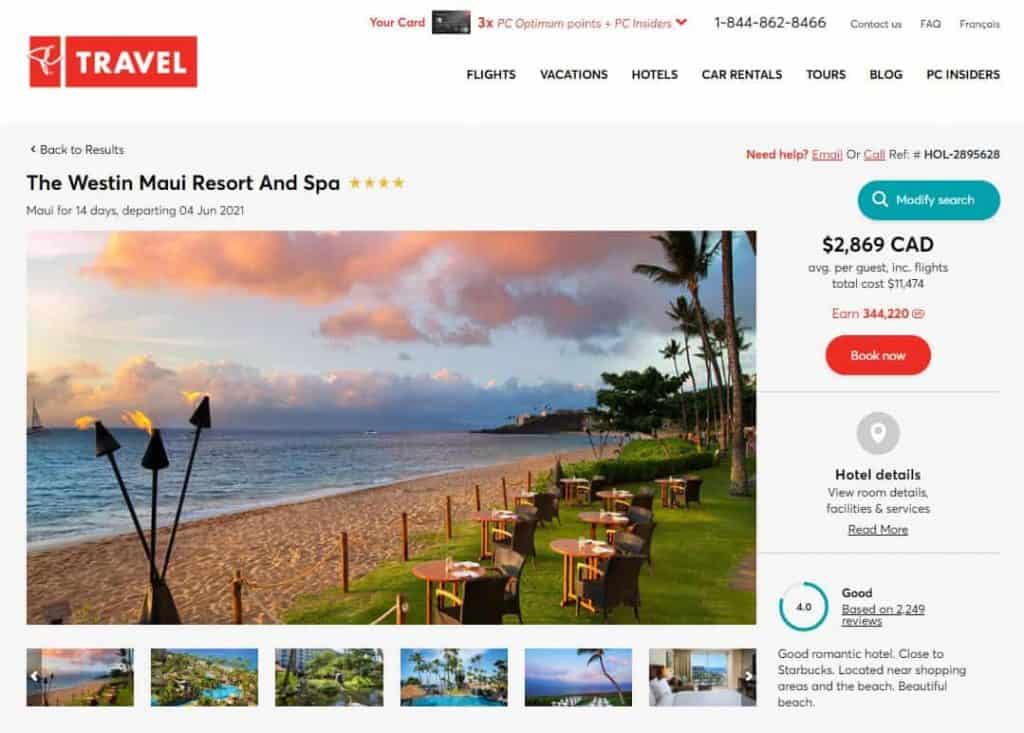The Travel.com homepage features the Westin Maui Resort and Spa, highlighting its luxury offerings on a dedicated page. At the top of the page, users can easily navigate through various categories such as flights, vacations, hotels, car rentals, tours, a blog, and the PC Insiders section. Essential contact information, including a phone number, fax number, and frequently asked questions, is readily available. 

The Westin Maui Resort and Spa is prominently displayed with a prestigious 4-star rating, accompanied by a price tag of $2,869 CAD for the stay. Detailed hotel information includes extensive ratings, reviews, and a gallery of high-quality images. Users can refine their search criteria or return to the previous results with just a click. For additional assistance, there's an option to email or call using the reference number provided at the top right of the page.

A brief description indicates an enticing offer: a 14-day stay in Maui, departing on June 4th, 2021, which may encompass a cruise and hotel package. To secure this deal, users can click the prominent red "Book Now" button. Additionally, this booking could earn substantial reward points, ranging from 300,000 to 440,000 credits.